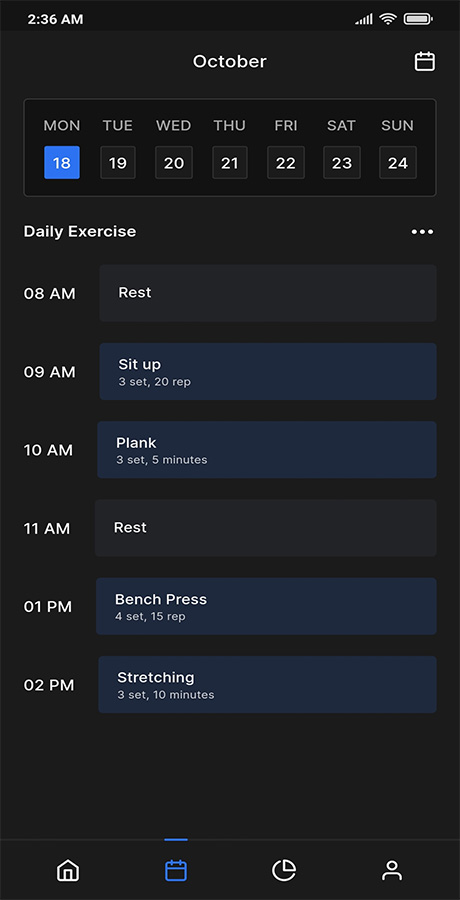Screenshot of Exercise Tracking App Interface

The screenshot captures the interface of an exercise tracking app on a cell phone screen with a sleek black background and contrasting white text, accented with blue highlights. 

**Top Bar:**
- **Time:** Displayed at the top left corner, reading *2:36 AM*.
- **Cell Phone Signal:** Full signal strength indicated by all four bars.
- **Wi-Fi Icon:** Showing active Wi-Fi connection.
- **Battery Icon:** Fully charged battery indicated by the full battery icon.

**Date and Days of the Week:**
- **Month Display:** Centered at the top is "October".
- **Days of the Week:** Just below the month, the days Monday through Sunday are listed, covering the dates from the 18th to the 24th of the month. 
- **Current Day Highlight:** Today’s date (e.g., *Thursday, 20th October*) is highlighted within a blue square with white text.

**App Content:**
- **Section Title:** "Daily Exercise" is prominently displayed.
- **Menu Option:** A clickable three-dot menu icon is situated to the right of the title.

**Exercise Schedule:**
- **8:00 AM:** Marked as a rest period indicated by the word "Rest" in a dark gray rectangular button.
- **9:00 AM:** Exercise listed as "Sit Up" with a routine of three sets of 20 reps.
- **10:00 AM:** “Plank” exercise noted, with three sets lasting five minutes each.
- **11:00 AM:** Another rest period indicated by the word "Rest".
- **1:00 PM:** "Bench Press" exercise, consisting of four sets of 15 reps.
- **2:00 PM:** "Stretching" session allocated, comprising three sets of 10 minutes each.